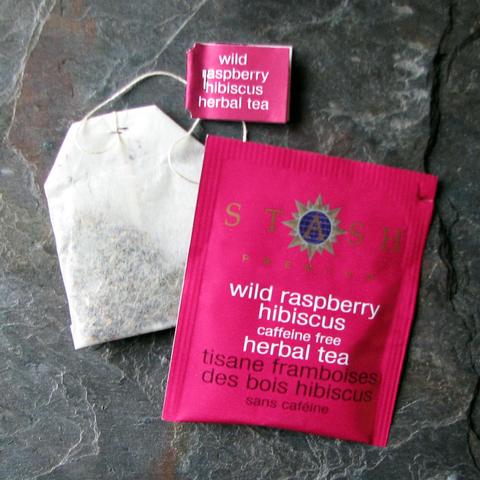This photograph showcases a standard white teabag to the left, filled with tea and featuring a reddish-purple square tag with white text that reads "wild raspberry hibiscus herbal tea." The teabag is connected to the tag by a string. Positioned to the right of the teabag is its corresponding plastic or paper pouch, sharing the same reddish-purple color. The pouch prominently displays the Stash logo at the top, which includes a turquoise and blue sunburst mandala pattern encircling the letter 'A'. Below the logo, in white font, it states "wild raspberry hibiscus caffeine-free herbal tea," followed by the French translation "Tisane Framboises de Bois Hibiscus sans caféine" in black font. Both items rest against a gray marble countertop, with the overall image presenting a clear and detailed depiction of the tea and its packaging.